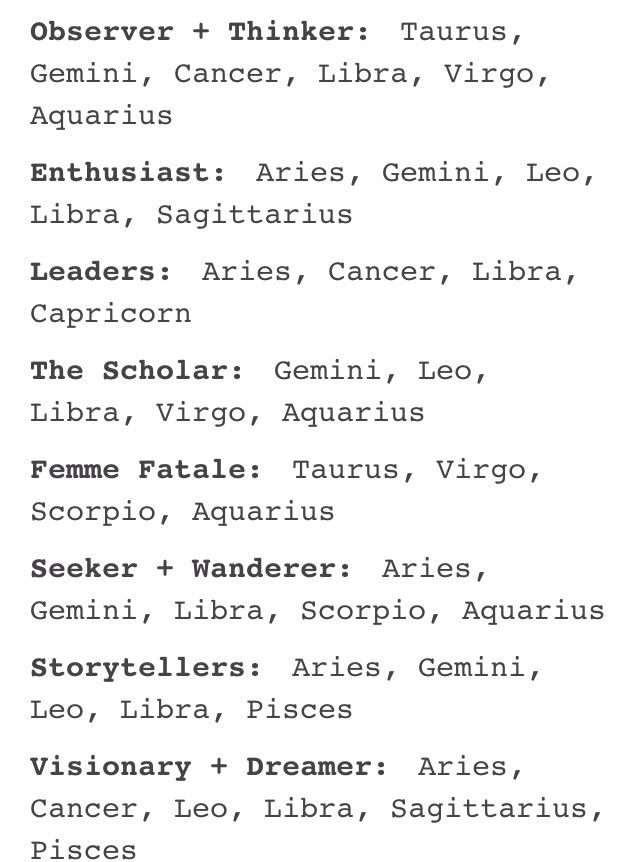The image features a white page with black and gray text detailing various horoscope archetypes associated with specific zodiac signs. At the top, the text reads "Observer plus Thinker," listing Taurus, Gemini, Cancer, Libra, Virgo, and Aquarius. Below, the category "Enthusiast" includes Aries, Gemini, Leo, Libra, and Sagittarius. The "Leaders" archetype contains Aries, Cancer, Libra, and Capricorn. "The Scholar" associates with Gemini, Leo, Libra, Virgo, and Aquarius. The "Femme Fatale" category lists Taurus, Virgo, Scorpio, and Aquarius. Under "Seeker plus Wanderer," the signs are Aries, Gemini, Libra, Scorpio, and Aquarius. "Storytellers" features Aries, Gemini, Leo, Libra, and Pisces. Lastly, "Visionary plus Dreamer" includes Aries, Cancer, Leo, Libra, Sagittarius, and Pisces. The text is presented on a plain white background, with varying thickness in the font, and repeatedly mentions the zodiac sign Libra.